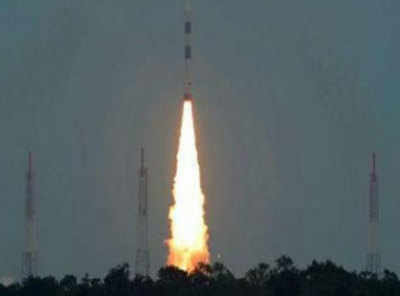The image showcases a rocket launching into a dusky sky, marked by shades of bluish gray, typical of either early morning or evening. The photograph is of low quality, appearing grainy and unprofessional. The silhouette of tall trees is visible at the bottom, along with three high, metal tower-like structures possibly supporting the launch. The rocket itself is white with two blue bands spaced along its body and is ascending straight up, leaving behind a dramatic trail of thick flames. The fiery trail transitions in color from a bright white at the rocket’s engines to pale yellow, rich yellow, and finally deep orange closer to the ground. The sky is clear, lacking clouds, and the predominant illumination comes from the rocket's propulsion flames.